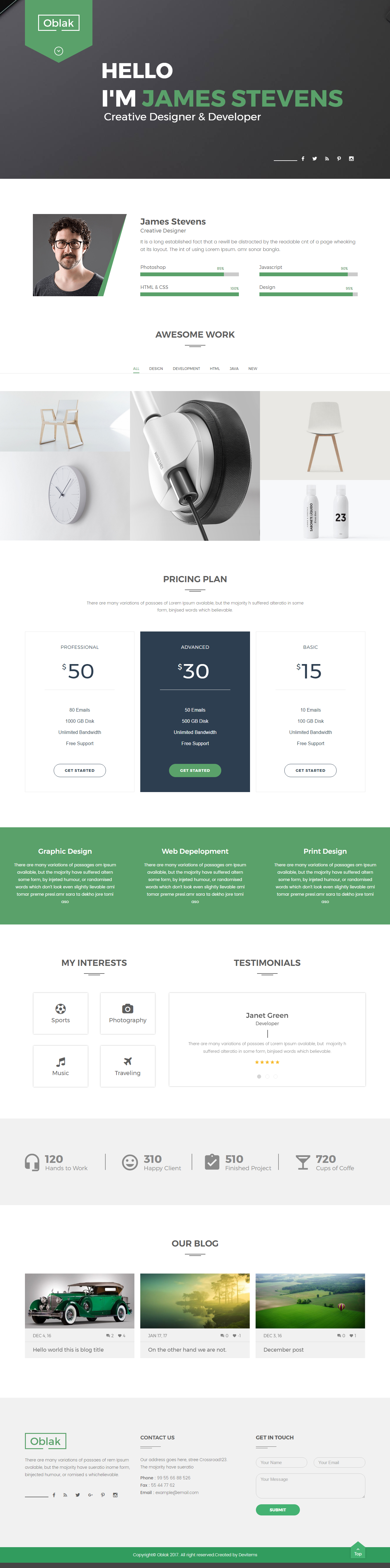A screenshot of a well-designed landing page introduces James Stevens as a creative designer and developer. The background is sleek black, giving the page a modern and professional look. At the top, "Hello, I'm" is boldly displayed in white, with "James Stevens" prominently featured in green, all capitalized. This text is followed by a subheading announcing his profession.

Below this introductory text, there's a professional headshot of James Stevens, accompanied by a detailed paragraph about him. Adjacent to the paragraph are two green bars placed side by side, enhancing the visual appeal. Beneath this section, the layout includes a row of three distinctive images: a clock paired with a chair, a stylish chair flanked by two drink cups, and an elegant light fixture.

Further down, the page showcases three promotional boxes with different color schemes: white, black, and white. They display pricing details, with the white boxes indicating $50 and $15, and the black box indicating $30. 

A larger rectangle near the bottom of the page contains three in-depth paragraphs, presumably elaborating on James’s projects, skills, or services. This is followed by a section divided into four areas titled "My Interests," providing an insight into his personal or professional passions.

Finally, a dedicated testimonials section features client feedback or accolades, framed by a gray box with four icons at the bottom, likely representing different social media platforms or contact methods, rounding off the comprehensive and engaging design of the landing page.